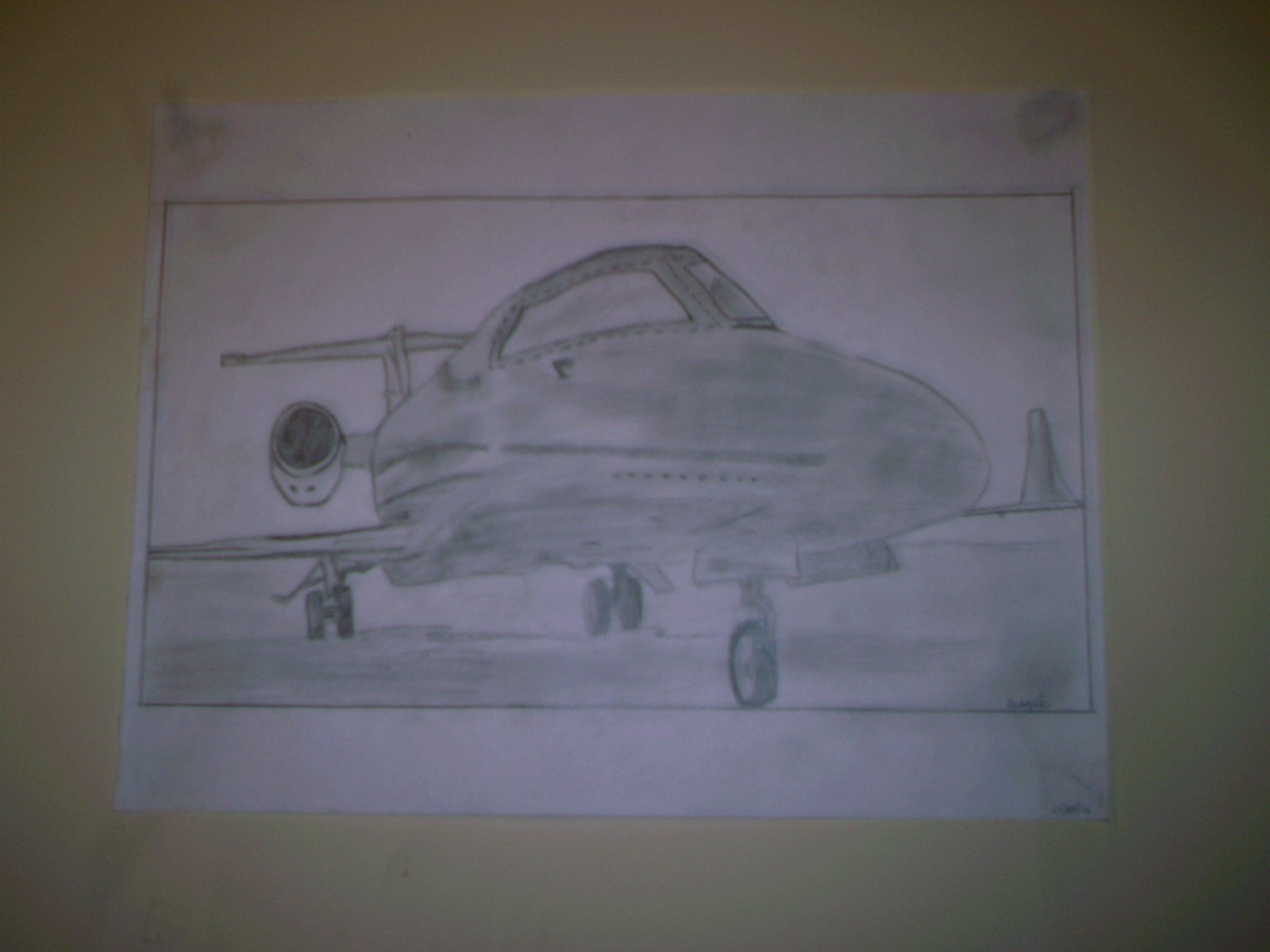This color photograph features a detailed pencil drawing of an airplane on a sheet of white paper against a dimly lit, dark yellowish background. The image appears grainy due to poor lighting conditions. The drawing includes a front-side view of the airplane, depicted in light grey pencil shading, with intricate details such as one of the airplane's windows, the right engine with a distinct round black center, and a portion of the tail. The ground beneath the plane is partially shaded in light grey as well. Above the drawing, two small dots are colored in at the top of the paper. To the left side, a faint outline of the wing can be seen, while on the right side, an ambiguous shape looms in the background, which could either be part of the other wing or a tall, narrow mountain. This detailed artwork captures the essence of an aircraft with a touch of ambiguity in its surroundings.